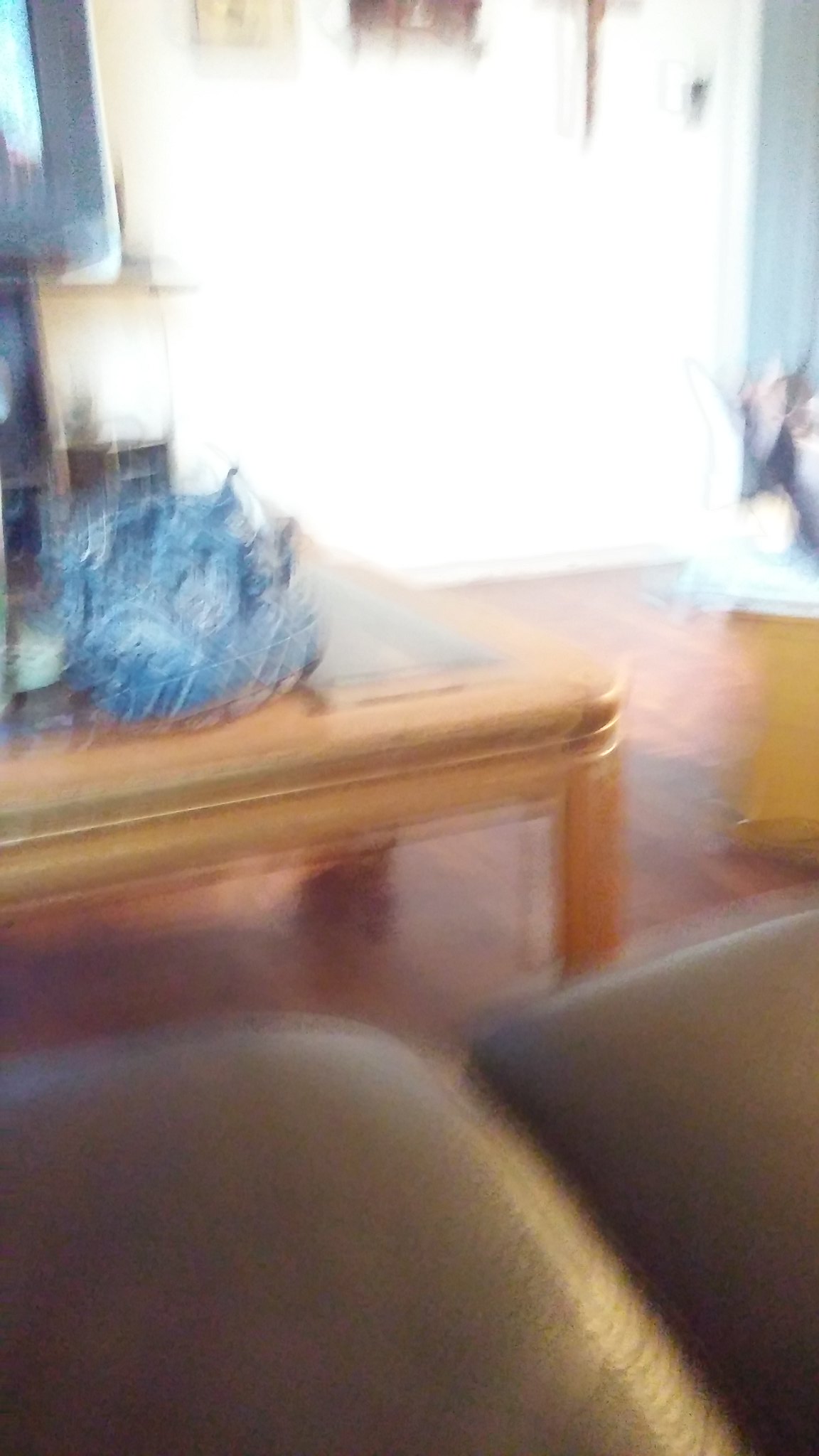This image captures a somewhat blurry view of a living room dominated by a large window in the center background, which floods the upper third of the picture with bright light. The intense brightness from the window obscures some details, creating a soft, ethereal glow. To the left of this illuminating window, a small section of a blue-painted wall is visible. At the base of this wall sits an ornament or decorative piece, although its specific details are unclear due to the blur.

Adjacent to the wall, there is a wooden coffee table resting on sleek wood flooring. This table prominently features a sizable, blue object on its surface, which appears to be a large stone, rock, or perhaps a mineral gem, adding an intriguing focal point to the scene. Further in the distance, a brown couch is situated against the far wall, contributing to the cozy and inviting atmosphere of the living room. Despite the blurriness, the layout and elements within the room suggest a warm and lived-in space.